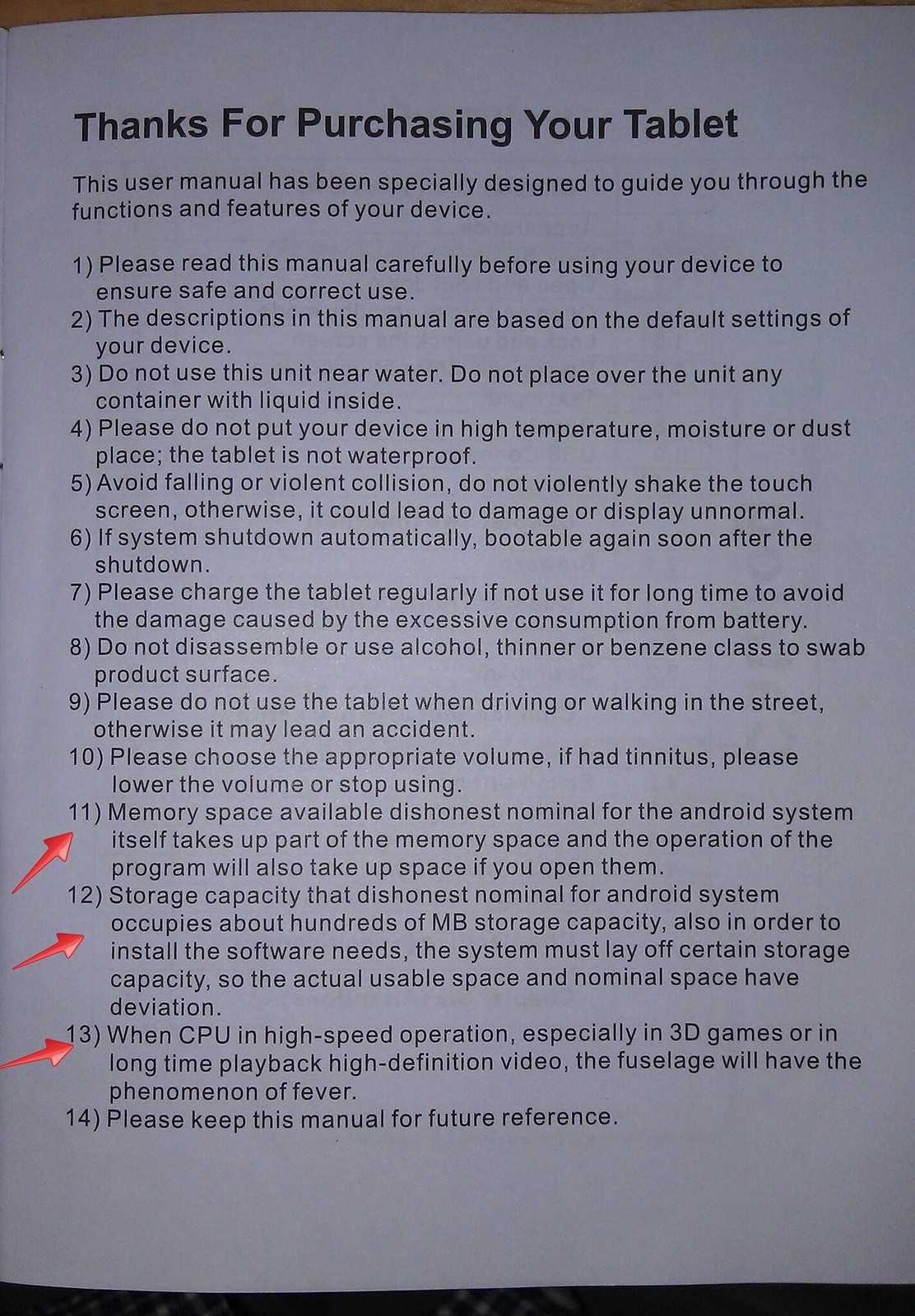The vertically aligned rectangular image depicts a page from a user manual, possibly part of a booklet, indicated by the slight downward curve on the left side. The page is titled "Thanks for Purchasing Your Tablet" in large black letters, left-aligned above smaller black text. Beneath the title, the text reads: "This user manual has been specifically designed to guide you through the functions and features of your device." Below this introduction, a numbered list from 1 to 14 is left-aligned, explaining essential safety and usage instructions for the tablet. Each number is followed by a right parenthesis and a couple of lines of description. Highlights include safety protocols such as avoiding water and high temperatures, proper handling, guidance on device memory and storage capacity, and maintaining battery health. Specifically, red arrows from the left side point towards numbers 11, 12, and 13, focusing on points about memory space, storage capacity, and high-speed CPU operations causing heat. The overall color scheme comprises black text on a white background, with red arrows, reflecting a standard informative style typical of product manuals.